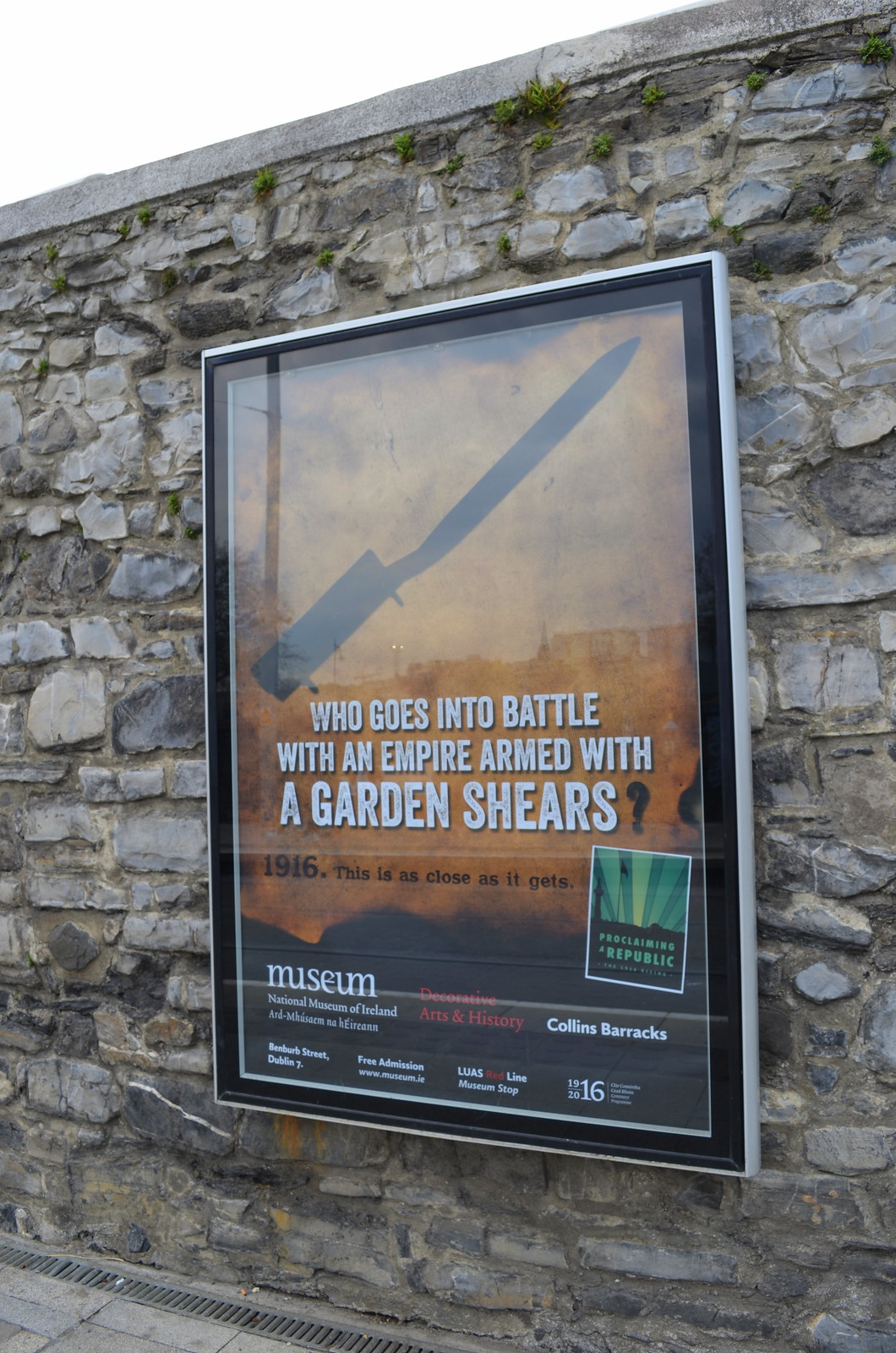The image depicts a stone wall made up of gray, black, and beige rocks, with a close-up perspective that highlights the texture as bumpy and held together by concrete. At the very top of the wall, some green moss and weeds can be seen growing between the stones. A poster is prominently displayed on this stone wall, encased in a silver frame with glass, which reflects the overcast sky.

The poster itself has an orange background and features a central silhouette of a blade or garden shears. Above the silhouette, in capital white letters, it reads: "Who goes into battle with an empire armed with garden shears?" Beneath this, there's the year mentioned, "1916," followed by the phrase, "This is as close as it gets."

Additional text at the bottom of the poster refers to the "Reclaiming a Republic Museum," along with the "National Museum of Ireland," emphasizing "Decorative Arts and History" at "Collins Barracks." There is also specific location information, including "Benburb Street, Dublin 7," and notes on "free admission," proximity to the "LuáS Red Line," and "Museum Stop," possibly indicating public transport directions.